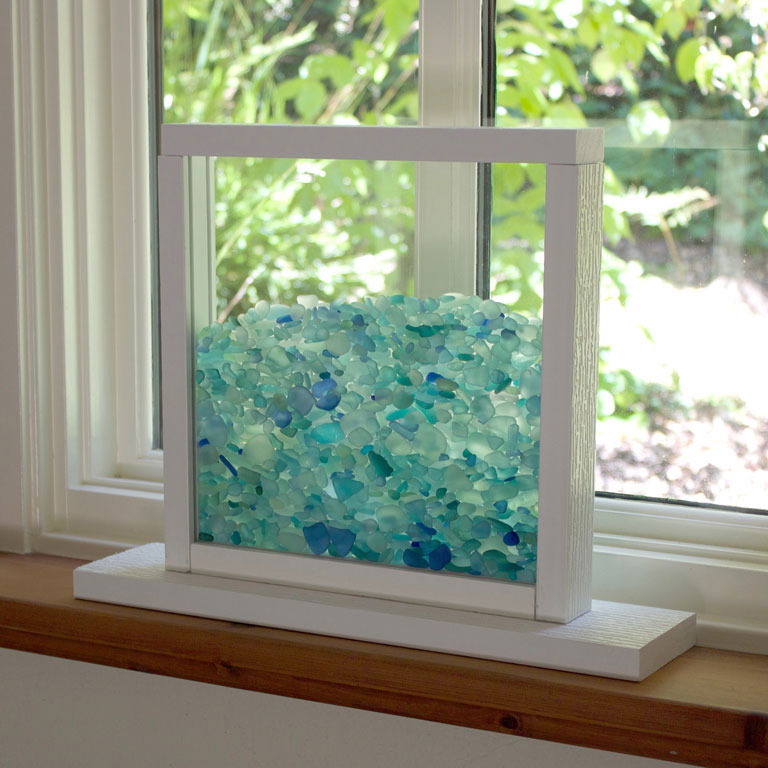A decorative piece of glass, framed in a white-painted wooden structure with shallow depth, is positioned on a windowsill in a bright, sunny room. This rectangular frame, featuring two panes of glass, is mounted on a stained wooden ledge next to a modern vinyl window. Inside the glass enclosure, a collection of crystals - predominantly in shades of light blue and green, with some darker blue and white stones - fills the space a little over halfway. The sunlight streaming through the window illuminates the varied shapes and sizes of the crystals, casting a gleaming reflection. Outside, a lush, green-leafed tree is visible, accentuating the serene and vibrant ambiance.